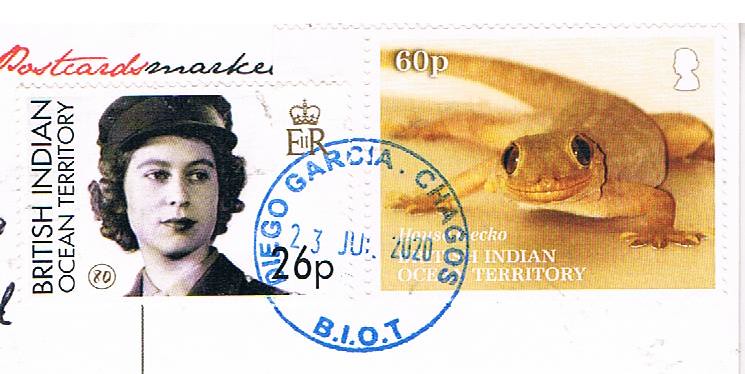This image features the upper half of a postcard adorned with two distinct stamps and a postmark. The first stamp, situated on the left, showcases a young Queen Elizabeth II, with the text "British Indian Ocean Territory" positioned beside her portrait. This stamp includes the crown symbol with the letters "ER" and is valued at 26 pence. Adjacent to Queen Elizabeth's stamp, on the right, is a vibrant 60 pence stamp depicting a charming gecko, its eyes appearing to focus directly at the camera, and labeled as a "House Gecko." Above these stamps, a blue ink postmark reads "Diego Garcia, Chagos, B.I.O.T., July 23, 2020," indicating the mailing date and location. A partially visible text at the top of the postcard likely identifies it as a "Postcards Marker," though the complete word is obscured. The postcard appears to be cut off, providing a glimpse into its journey from the British Indian Ocean Territory.